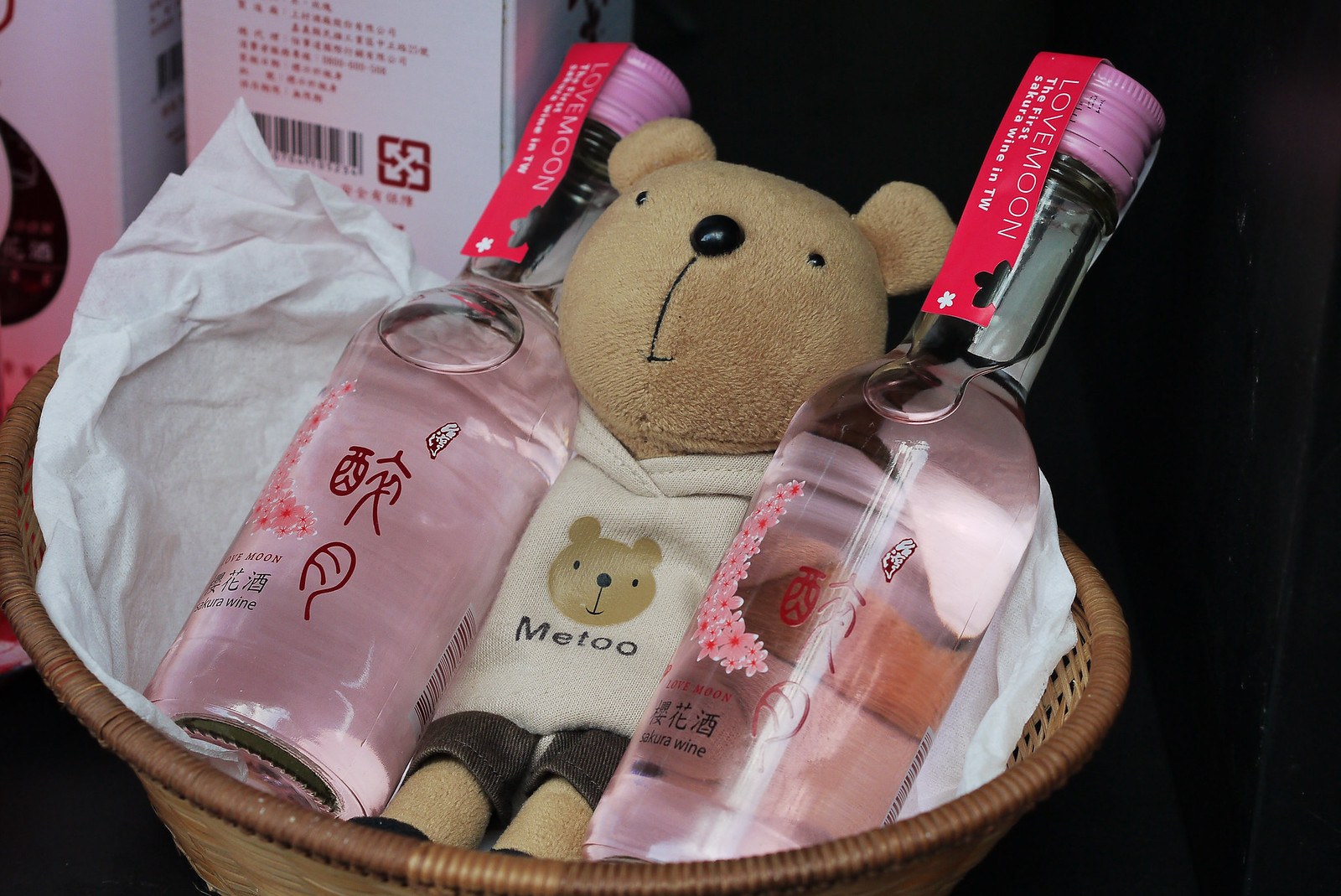The photograph displays a rectangular arrangement with a predominantly black background. In the foreground, there's a brown wicker basket filled with white tissue paper, placed at an angle that makes the left side higher than the right, which extends towards the lower right corner without reaching it. In the center of the basket sits a small brown teddy bear dressed in a white shirt with a printed bear face and the text "ME TOO" underneath. The teddy bear also wears dark brown shorts and brown shoes, making it an endearing focal point. Flanking the bear on either side are clear bottles with pink liquid inside, featuring pink caps and decorated with pink and white floral designs. These bottles have red labels with white text, "LOVE MOON," and additional smaller labels featuring the words "Sakura Wing" and "NTW." In the upper left corner of the image, partially visible pink boxes with red Asian writing add an extra layer of detail to this charming gift basket composition.